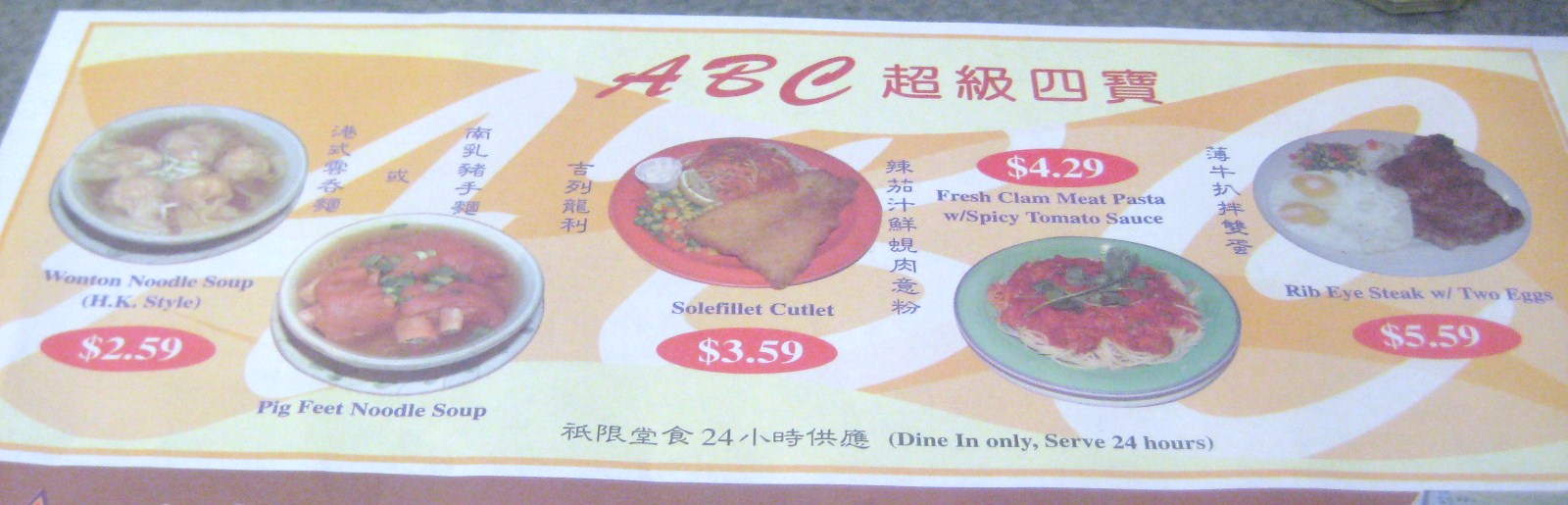This is an image, likely seen in an Asian restaurant, showcasing a promotional sign or paper advertisement displaying a variety of meal offerings. The sign prominently features the text "ABC" both in English and an Asian script, and includes vibrant images of different dishes with detailed descriptions and prices. 

1. **Wonton Noodle Soup** - Priced at $2.59, this dish is depicted as a soup-based meal with floating dumplings, highlighting the traditional wonton noodle soup.

2. **Pig Feet Noodle Soup** - This dish showcases visible pink pig feet immersed in the soup, catering to those who appreciate this unique and flavorful dish.

3. **Filet Cutlet** - Accompanied by a colorful arrangement of side vegetables in green, yellow, and orange hues, this cutlet is served on a red plate with a cup of sauce, ideal for those seeking a balanced meal.

4. **Clam Meat Pasta with Spicy Tomato Sauce** - This pasta dish is topped with fresh clam meat parts and a spicy tomato sauce, offering a seafood twist on a classic pasta.

5. **Rib Eye Steak with Two Eggs** - Presented on a white plate, this hearty meal includes a rib eye steak paired with two eggs and garnishments, catering to those with a taste for a classic and robust entrée.

The sign effectively presents a diverse range of dishes, appealing to a variety of palates and preferences.